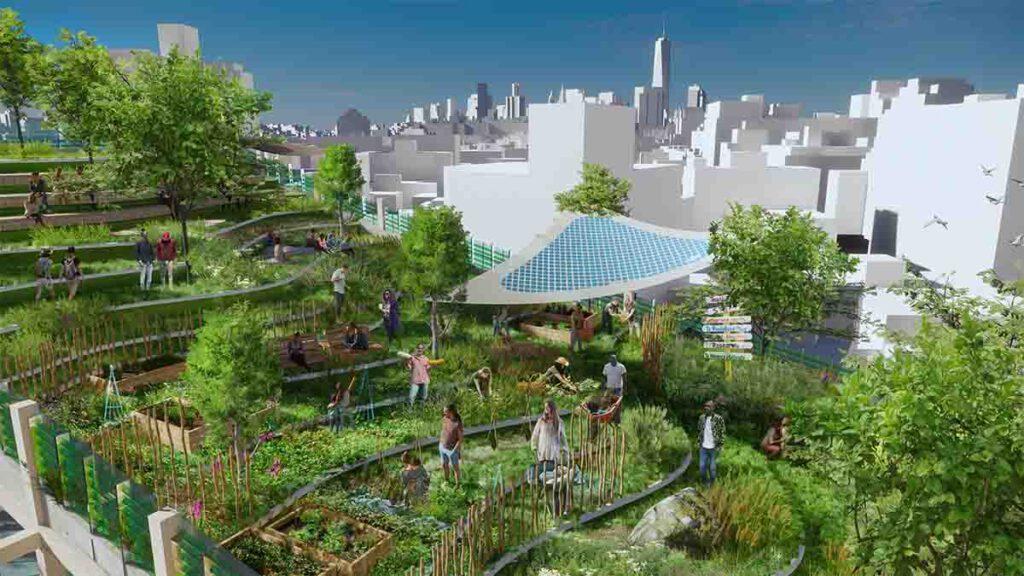The image depicts a futuristic and clean-looking cityscape, characterized by sleek white and silver buildings that dominate the background against a clear blue sky. It appears to be a computer-generated rendering, showcasing a stunning blend of urban development and green spaces. In sharp contrast to the high-rise skyline, the foreground features an elevated, verdant urban oasis, resembling the repurposed concept of New York's High Line. This area is lush with trees, flowers, and various types of gardens, including vegetable plots within wooden square beds.

People are actively engaged in this communal space, either tending to their gardens or relaxing. There are several notable elements, such as a white canopy with a blue roof, a white wall on the bottom left, and a few signposts with directions. One particularly interesting feature is a tent equipped with solar panels, adding a touch of sustainable technology to the scene. Additionally, wheelbarrows can be seen as people go about their farming activities. Overall, the image highlights a harmonious blend of modern urban architecture and sustainable, green living spaces.